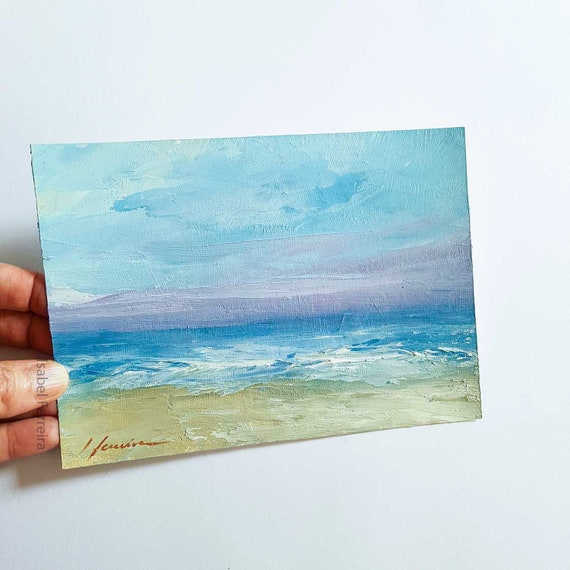In a studio or home setting, a left hand is prominently holding a small watercolor painting of a seaside landscape against a white background. The artwork vividly depicts a beach scene with a layered sky that transitions from green at the top, blue below it, and subtle grey near the horizon. Below the sky, a grey mountain gives way to a blue sea featuring white waves gently lapping at a light sandy shore. The right side of the shore is accented with streaks of white paint. The hand's thumb is clearly visible, securing the postcard-sized painting which conveys the tranquility of a sunset, with some lavender hues blending into the expansive blue sky.